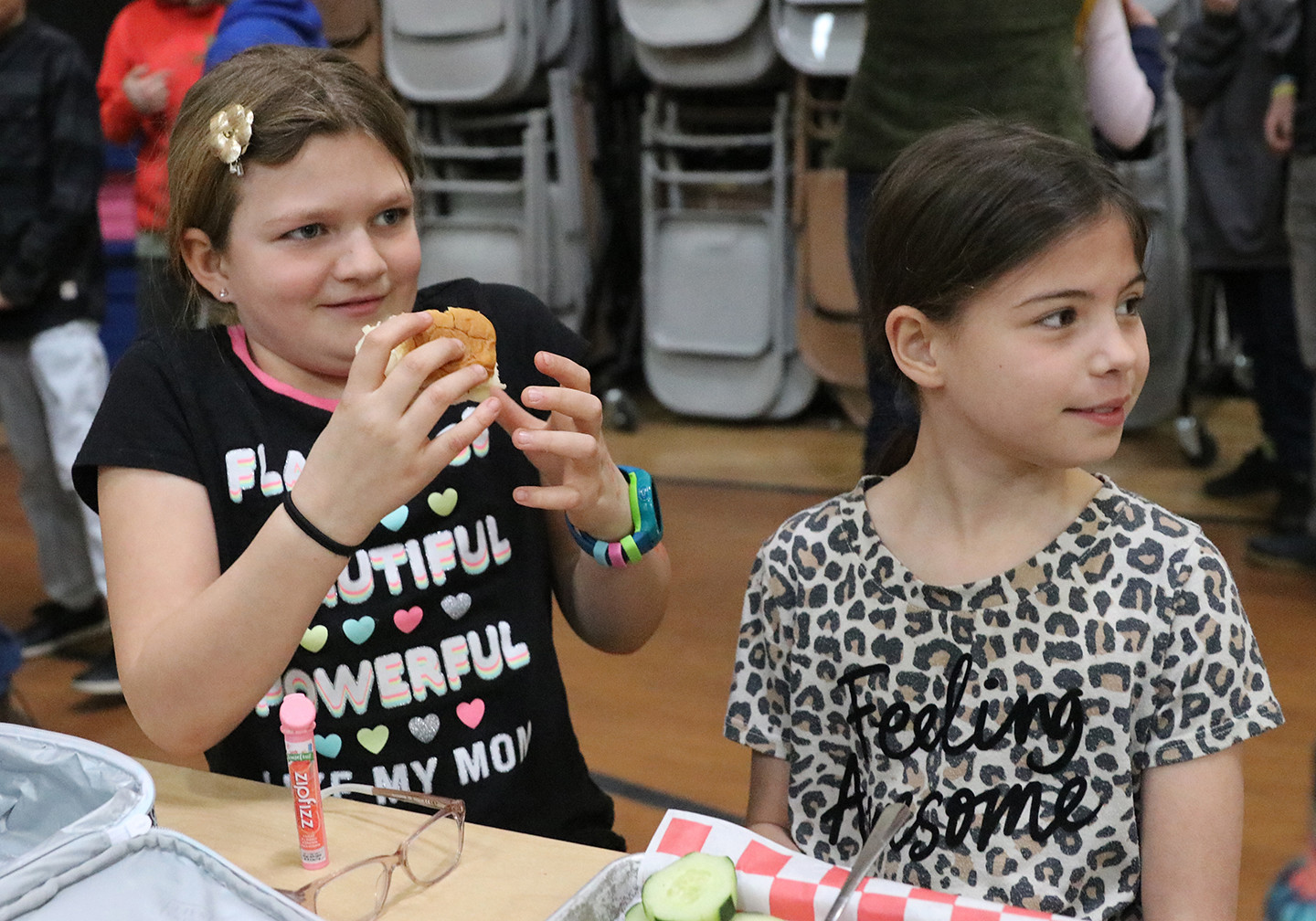In a bustling cafeteria, two young girls, both appearing to be around ten years old, are seated at a light brown wooden table, engrossed by something off to the right. The girl on the left is dressed in a black soft-sleeve t-shirt adorned with vibrant, colorful hearts and the empowering words, "Beautiful, powerful, like my mom." Her brown hair, pulled back into a delicate ponytail, is accentuated by a golden flower-shaped hair clip and a single earring glistens in one ear. She clutches a half-eaten bun in her hand, and a colorful watch featuring hues of blue, lime green, and pink graces her wrist. In front of her lies a soft padded lunchbox, decorated with pastel pink glasses and an item labeled "Whipsbiz." 

The girl on the right dons a brown soft-sleeve t-shirt with a leopard print and the phrase "Feeling Awesome" scripted in black cursive. She too has her hair tied back in a small ponytail. Before her is a tray lined with red and white paper, holding slices of cucumber, and the handle of a utensil can be seen peeking out. A lively scene unfolds behind them, with several chairs stacked together and the lower bodies of other children and adults visible, set against the backdrop of a wooden gym floor. This vivid image captures a moment of their midday meal amidst the school's vibrant lunchtime atmosphere.